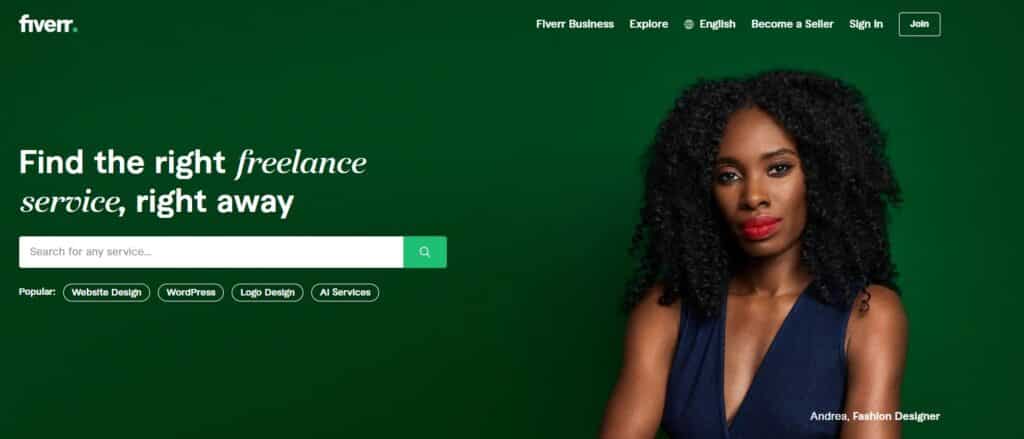The image, intended for a Fiverr promotional webpage, prominently features the Fiverr logo in the upper left corner set against a green background. All text on the page is rendered in white. The right side of the header displays navigation options, including "Fiverr Business," "Explore," "English," "Become a Seller," "Sign In," and "Join."

Dominating the left side of the page, the phrase "Find the Right Freelance Service Right Away" is prominently displayed. Below this, a search box with the placeholder text "Search for Any Service..." features a magnifying glass icon on its far right. Directly beneath, a list of popular search categories is mentioned: "Popular," "Website Design," "WordPress," "Logo Design," and "All Services."

In the bottom right corner, overlaid on a photograph of a young, smiling African-American woman with curly shoulder-length hair and red lipstick, the text reads "Andrea, Fashion Designer." The woman, who faces the camera with a slight smile, wears a gray top and no visible jewelry. The photograph crops her just above the elbows, leaving the rest of her attire and background to the imagination.